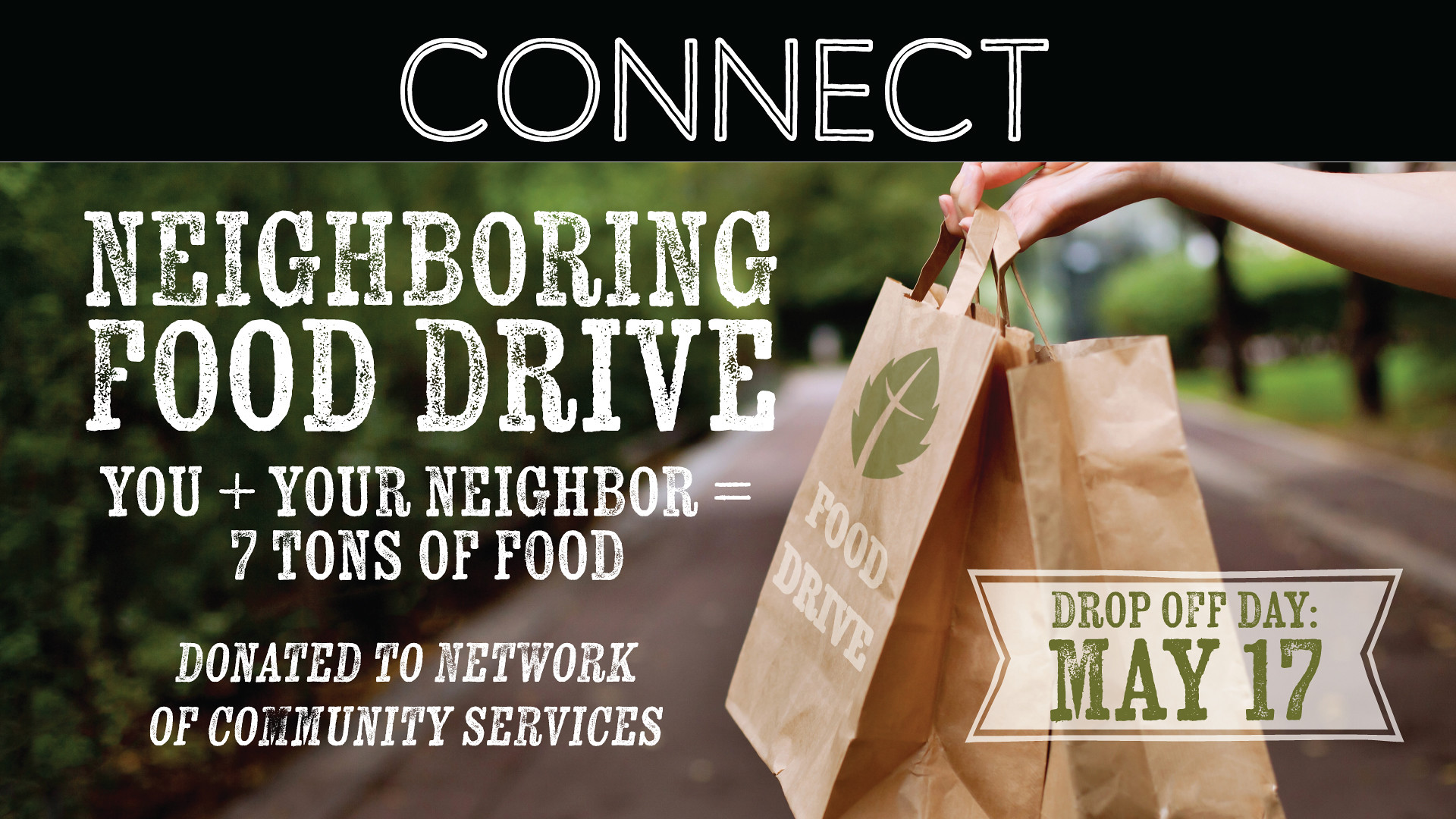This advertisement for a food drive features a top black rectangular banner with the word "CONNECT" in large white letters, accented with a touch of gray inside each letter. Below, the image showcases a scenic street backdrop with abundant greenery, especially on the left side of the frame. In the foreground, a woman's arm extends into view, holding two brown paper bags marked with "FOOD DRIVE" and adorned with a green leaf icon. The left side of the advertisement features white text detailing the event: "Neighboring Food Drive" and the impactful slogan "You plus your neighbor equals seven tons of food donated to Network of Community Services." A white rectangular section in light green at the bottom right announces the "DROP OFF DAY MAY 17."